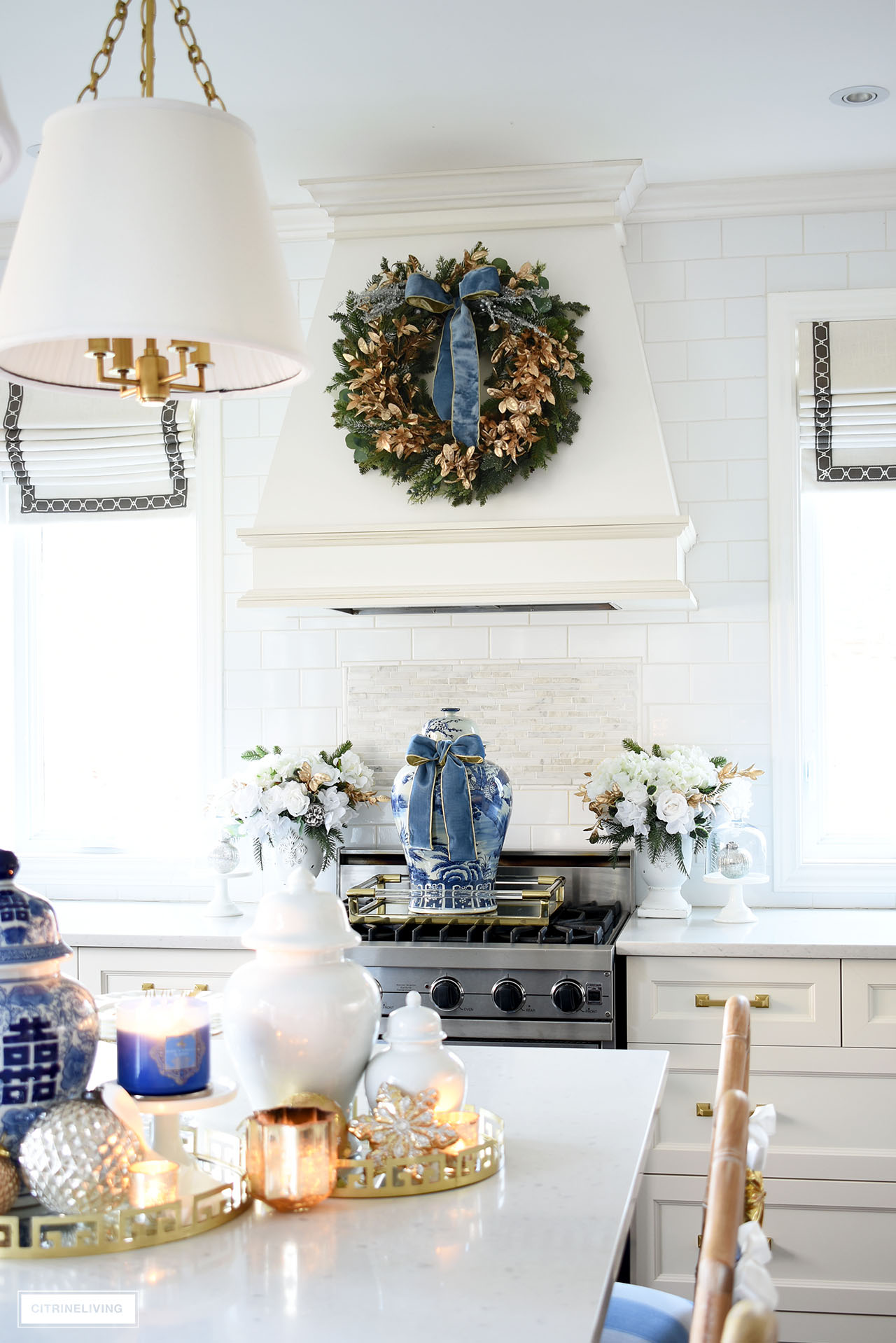The photograph captures an elegantly decorated, bright white kitchen set for Christmas. The centerpiece of the image is a silver gas stove adorned with a blue and white vintage teapot, situating beneath a sophisticated white vent hood. Affixed to the vent hood is a striking green Christmas wreath embellished with gold-patterned leaves and crowned with a coordinating blue bow. Flanking the stove, there are charming pots of white flowers situated before two windows fitted with white blinds edged in blue.

In the foreground, a polished gray kitchen table or counter effortlessly pulls the room together. On the table lies an array of holiday ornaments: white Christmas balls, a white candle in a blue cup, a gold cup, and a blue and white vase, all harmoniously reflecting the blue and white theme seen throughout the kitchen. To the top left of the image, a white chandelier featuring gold-bottomed light fixtures adds an extra touch of elegance. The overall ambiance of the space is clean, neat, and serene, exuding festive cheer through its meticulous decor and cohesive color palette of white, blue, and gold.